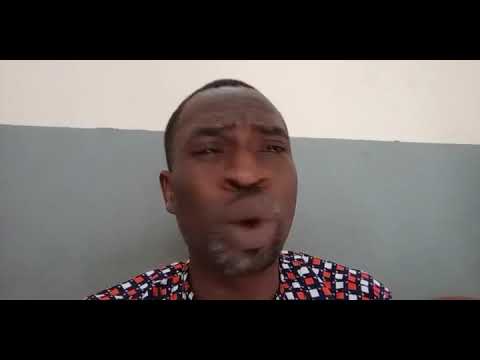The image captures a young black man, likely in his 20s or 30s, standing directly in the center of the frame. The photograph shows him from the shoulders up, revealing his very short black hair and a black and gray goatee. His facial expression suggests he might be talking or reacting to something, with his slightly open mouth and wincing eyes, almost as if he's in mild discomfort. He has prominent features, including large lips and a significant nose.

The man is wearing a checkered collared shirt, featuring a pattern of red, white, and black squares, giving it a bold and distinctive appearance. The background consists of a two-tone wall: the lower two-thirds is gray, while the upper third is white. Additionally, the image is bordered by horizontal black bars at the top and bottom. The overall scene gives the impression of a candid moment captured amidst a minimalist setting.